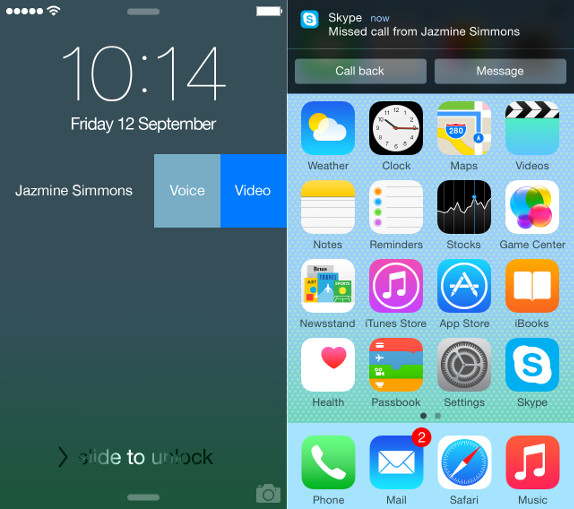This image consists of two side-by-side smartphone screenshots. 

On the left, we observe a lock screen with a gradient background that transitions from bluish-gray at the top to subtle green at the bottom. Centered prominently at the top is the time, displayed in large white numerals reading "10:14". Directly below this, also in white, is the date, "Friday, 12 September." At the top left corner, the Wi-Fi icon is visible alongside five white dots, indicating signal strength. The top right corner features a fully charged battery icon, also in white. Beneath the date and time, the name "Jasmine Simmons" is displayed in white text. To the right of the name are two buttons labeled "Voice" and "Video", colored light blue and a medium blue respectively. At the bottom of the screen, instructions to "slide to unlock" are visible, marking this as a lock screen.

The right screenshot shows the home screen, which features a light blue background. The screen is organized into five rows and four columns of app icons. The visible apps include Weather, Clock, Maps, Videos, Notes, Reminders, Stocks, Game Center, Newsstand, iTunes Store, App Store, iBooks, Health, Passbook, Settings, Skype, Phone, Mail, Safari, and Music. Each app is represented by its distinctive icon within a small square.

This detailed visual description conveys a typical smartphone user interface with a blend of personal and standard features.